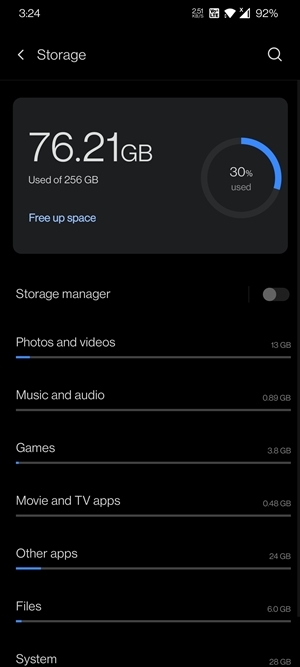This image is a cell phone screenshot displayed in portrait mode, showing a storage overview. The background is predominantly black, with a dark gray section for the main content. At the top of the screen, the upper left corner displays "324," and the upper right corner shows the battery level at 92%. Below this, a row features a back arrow, the word "Storage," and a search icon.

The main section under "Storage" reveals that 76.21 GB of the available 256 GB is used, indicating 30% of the total capacity. This usage is visually represented by a blue segment within a gray circle. A "Free up space" option is highlighted in light blue, suggesting the possibility of optimizing storage further.

The detailed breakdown includes:
- Storage manager: toggled off.
- Photos and videos: 13 GB (a small blue segment).
- Music and audio: 0 GB.
- Games: 3.8 GB (a small blue segment).
- Movies and TV apps: 0 GB.
- Other apps: approximately 24 GB (a significant blue segment).
- Files: 6.0 GB.
- System: not specified in detail.

This image provides a clear summary of the device's storage usage, indicating most data is consumed by apps and files, with substantial space remaining available.